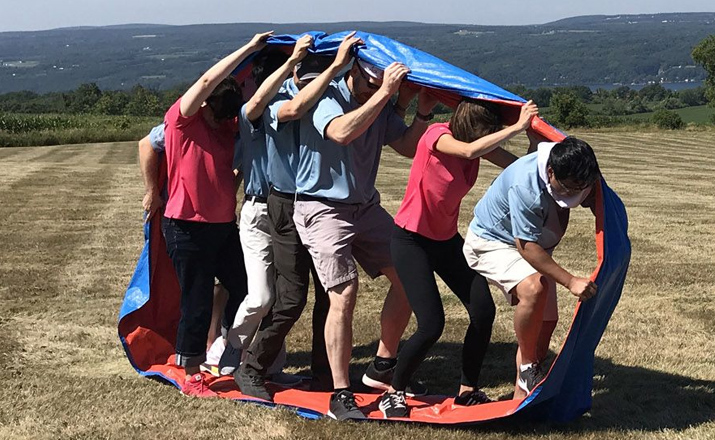The image captures a group of seven people engaged in a team-building exercise in a field, standing on a large, elastic, ring-shaped mat. The mat is colored blue on the underside and red on the top, the side they are all holding. The participants are mostly men dressed in blue shirts, with two women in red shirts. They are positioned in a line, walking together with the mat moving below them and over their heads. The person at the front is bent over significantly more than the others, gripping the mat tightly, while the rest maintain their hold with slightly bent knees. The field below them is covered in brown, dry grass, contrasting with the green grass, shrubs, and a bit of water visible in the distance. The backdrop includes verdant hills and green trees under a clear sky, suggesting an outdoor, possibly corporate event focused on building teamwork and camaraderie.